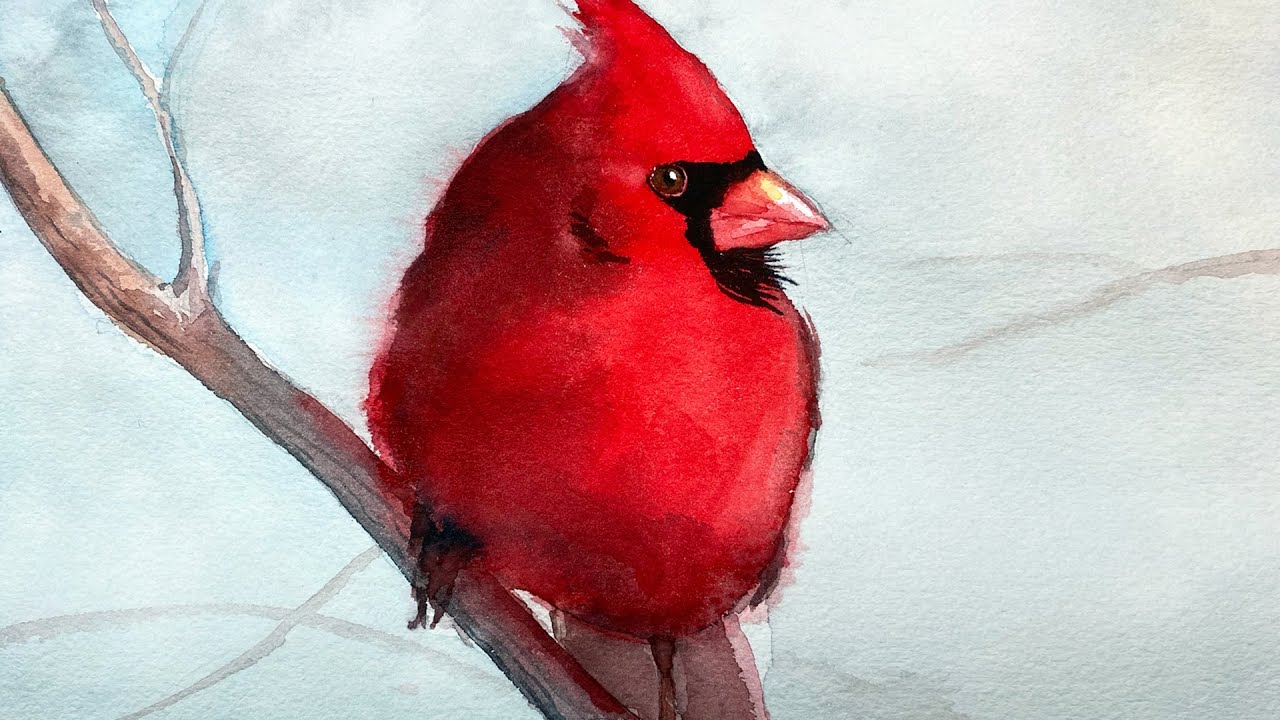This watercolor painting features a striking red cardinal with a black face, perched on a tree branch that extends in a sideways V pattern from the upper right side. The cardinal's wide body and pointed crest are vividly captured, with its head turned right, showcasing its short, orangish-pink beak and blackish-red claws. The textured background, intended to represent the sky, blends light gray, subtle browns, and patches of blue, adding depth. The large branch extends from the upper left side, with a smaller branch splitting off. Additional branches and limbs are faintly visible in the background, adding layers to the composition.